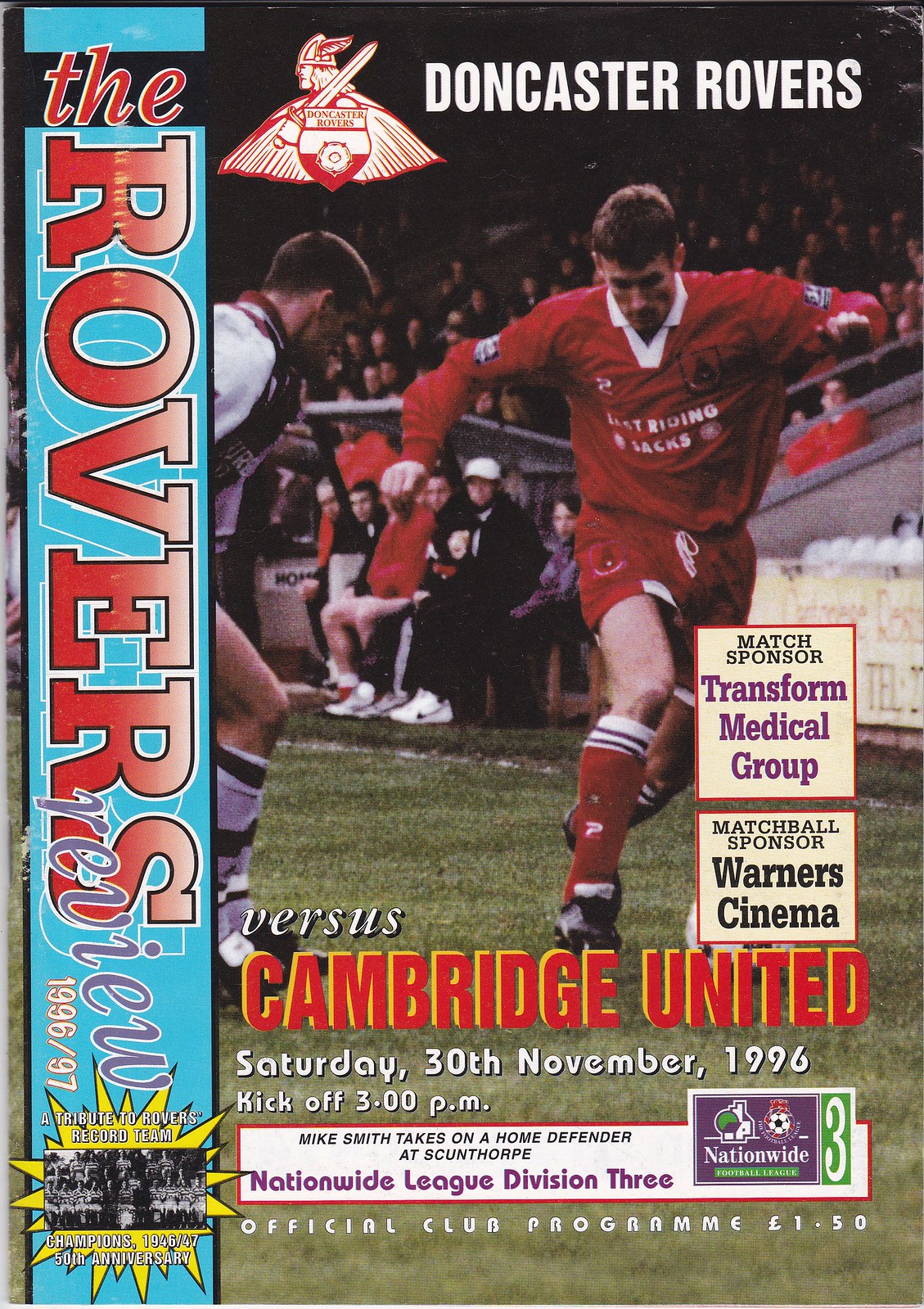This image is the front cover of an official club program for the Doncaster Rovers football (soccer) club from the 1996-1997 season, priced at £1.50. The cover features a tall, rectangular layout with a photograph prominently displayed. In the image, two players are seen on a green football field; the player in the foreground, wearing a red and white long-sleeved shirt, red shorts, and red socks, is about to kick a soccer ball. He has white skin and brown hair. Close by, an opposing player, wearing a white and red uniform, approaches him. The background shows a crowd of spectators watching the game. The top of the cover displays the red and white Doncaster Rovers logo, which resembles a Viking holding a shield, next to the text "Doncaster Rovers" in large white letters. Below the main image, the text reads "Cambridge United" in red letters, indicating the opponents of the match. Additional information on the cover includes the match details: "Saturday, 30th November 1996, kick-off 3.00 pm." The program also mentions match sponsors Transform Medical Group and Warner Cinema. On the left side, in a vertical orientation, is the text "The Rovers Review." The top right corner of the cover appears to be slightly scuffed, adding an element of wear to this historical program.